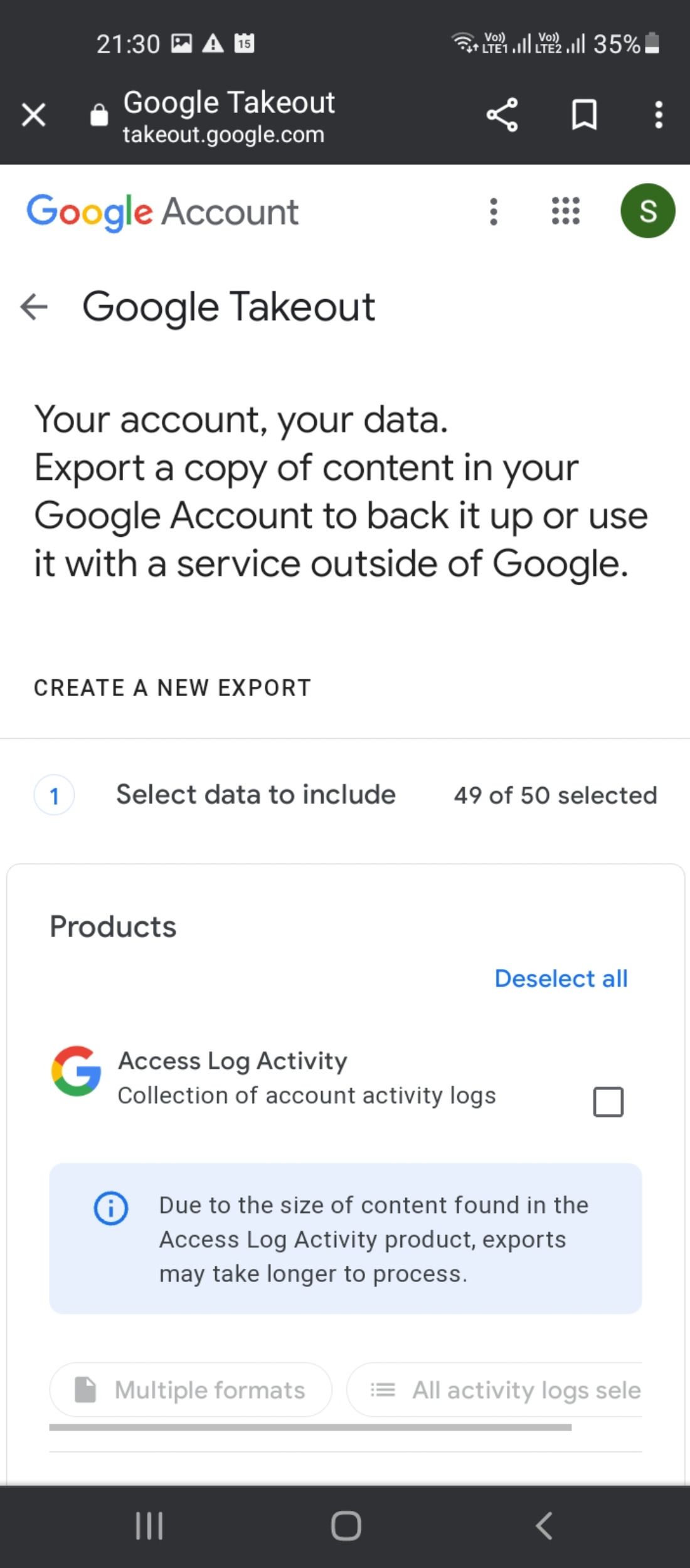### Screenshot Description of Google Takeout Interface

At the top, there is a header with a dark gray background featuring several traditional icons. On the top left, the time is displayed as "21:30" in white. Toward the top right, there is an image icon followed by a white triangle with a dark gray exclamation point, indicating a cautionary warning notification. Next to this is a white calendar icon marked with "15" in its center. Below this, towards the left, there is a white "X," suggesting the window has been maximized to landscape mode. 

Towards the right side of the header, there is a white padlock icon. Adjacent to this, "Google Takeout" is displayed in a basic sans-serif font. Beneath it, in a smaller white font, it reads "takeout.google.com." To the right of this, there is a shape resembling a triangle missing its bottom, with a white circular outline at each point, typically indicating a share button. Further right, there is a white bookmark outline, followed by three white dots suggesting a dropdown menu.

Below the dark gray header, the interface transitions to a white rectangular background. On the left side, the traditional colorful Google logo is displayed. To the right of the logo, "Account" is written in medium gray. To its right, there are three grey dots, followed by nine smaller dots forming a square shape. Further right, there is a dark green circle with a white "S" in the middle, presumably representing a user profile.

Underneath this section, towards the left, there is a gray arrow pointing left, indicating a navigational option to go back to the previous screen. To the right of the arrow, "Google Takeout" is written in a rounded sans-serif font in black.